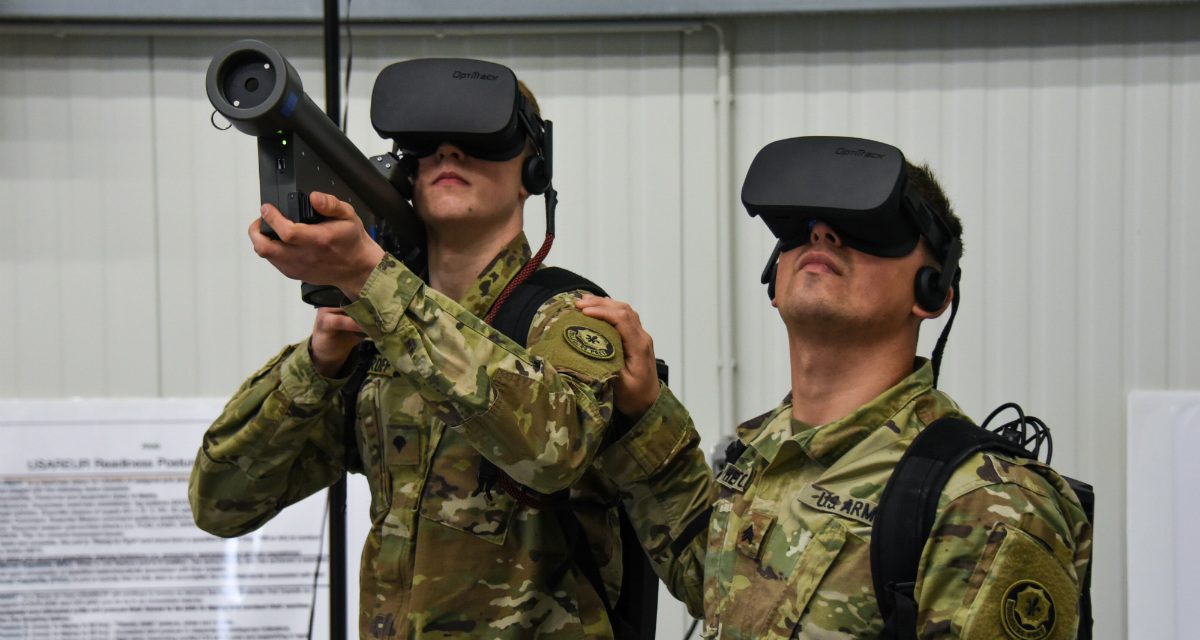In this detailed outdoor image, two young men are standing side-by-side in front of a white building with vertical siding. Both are dressed in U.S. Army camouflage uniforms that feature the U.S. Army insignia on their shoulders and various patches on their sleeves. They are wearing VR masks, which have large visors covering their eyes and partially their noses. The man on the left is holding a sizable, rocket-looking gun, reminiscent of a bazooka, which is part of their VR simulation. His arm is resting on the shoulder of the other man, possibly for stability. The signage is present on a fence to the left but is too small to read. Both men appear deeply engaged in the VR experience, completely absorbed in their simulated environment.